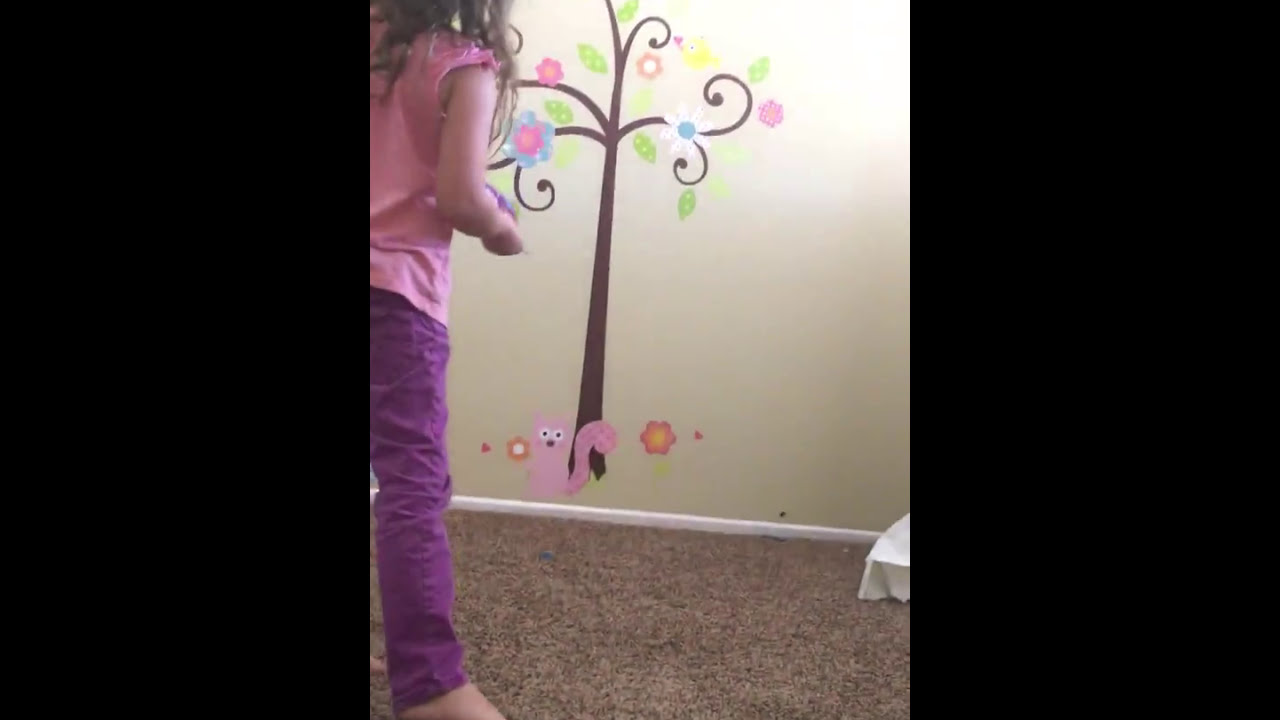The image captures the wall of a child's room adorned with whimsical decals. A simplified brown tree with curly branches and six or seven small squirrels, and decals of leaves and flowers against a tan wall create a playful scene. At the base of the tree sits a little pink squirrel with white eyes, surrounded by flowers. The left and right edges of the image are framed by thick black rectangle borders. A little girl stands barefoot on the tan carpet, wearing a short-sleeved pale pink shirt and purple jeans. She has long brown hair hanging below her shoulders and is partially cut off from the image, with her back turned to the camera as she looks at the decorated wall. Notably, she appears to be holding something in her hand.